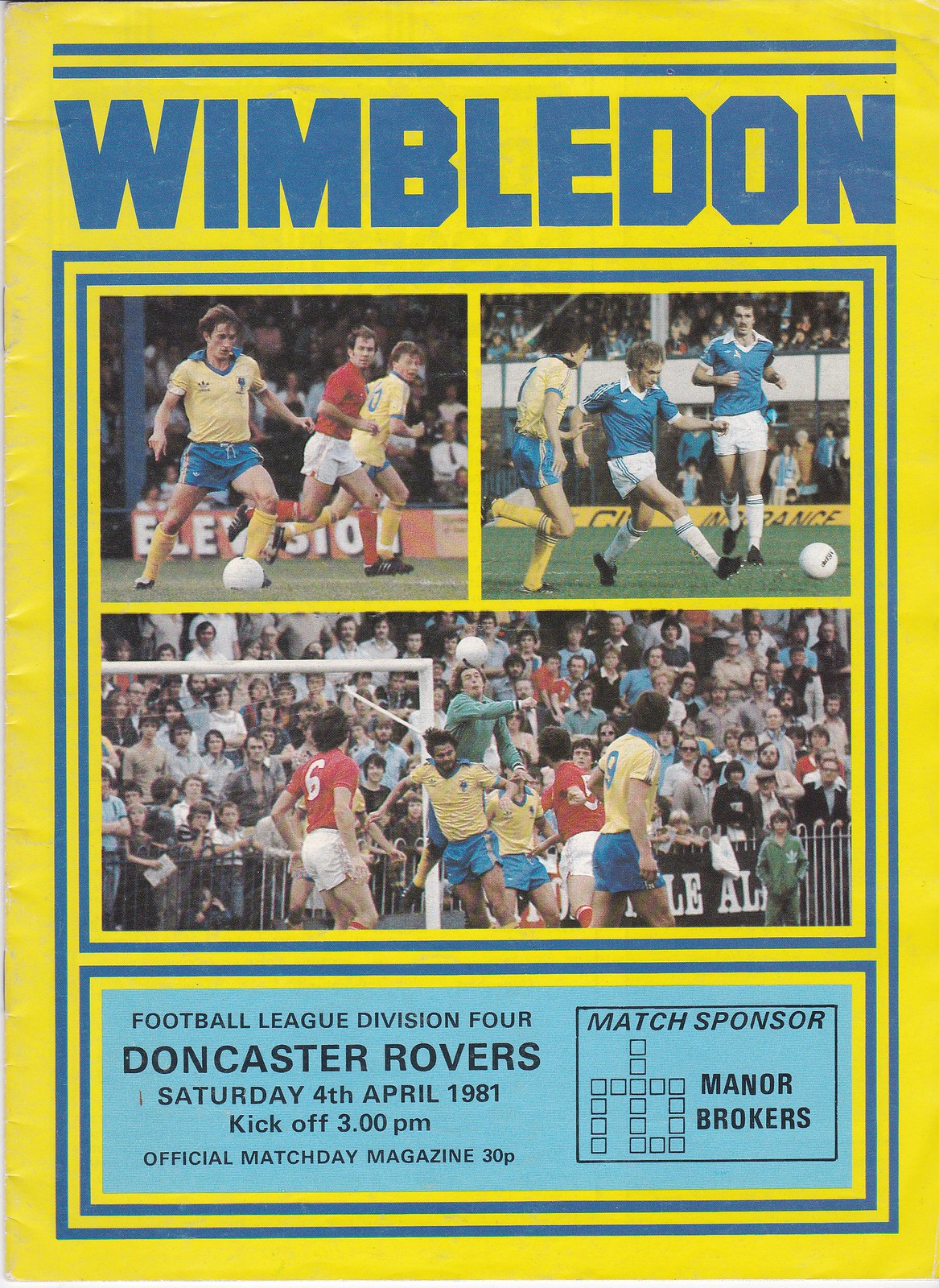This is a detailed photograph of a vintage Wimbledon Football Club magazine cover from 1981. The background of the magazine is a vibrant yellow, bordered in blue, with "Wimbledon" emblazoned in big, bold blue letters at the top. 

Prominently displayed in the center are three color action shots of Wimbledon players engaged in gameplay, capturing dynamic moments on the field. These still photographs add a lively touch to the cover.

At the bottom of the cover, detailed event information is listed: "Football League, Division 4, Doncaster Rovers," followed by "Saturday, 4th April 1981, Kickoff, 3 p.m." Additionally, it states "Official Match Day Magazine, 30p," and mentions the match sponsor, "Manor Brokers."

The colors featured in the image include yellow, blue, red, white, green, tan, black, and gray, making for a striking and attention-grabbing design. The overall appearance and layout suggest this is an official match day program, typically handed out to attendees at the game.